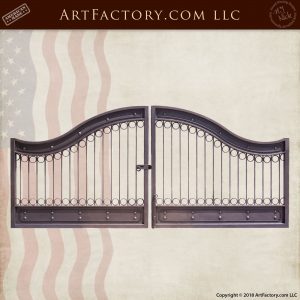The image appears to be an advertisement or a catalog cover featuring a photograph of a metal gate. The background is primarily off-white with a faint, vertically positioned American flag on the left side, showcasing its blue field with white stars and several wavy red and white stripes. The gate, square in shape, dominates the image and is characterized by its grey metallic bars, two-part structure, and an arched design at the top. The gate is adorned with several decorative features, including vertical spikes with small circles at their tips. There is a latch in the middle where the two parts of the gate meet. At the very top of the image, a brown rectangular banner displays the text "ArtFactory.com LLC" in light brown font. Additional elements include an unreadable stamp-like mark on the upper left and a round stamp on the right, adding to the advertisement's intricate design.